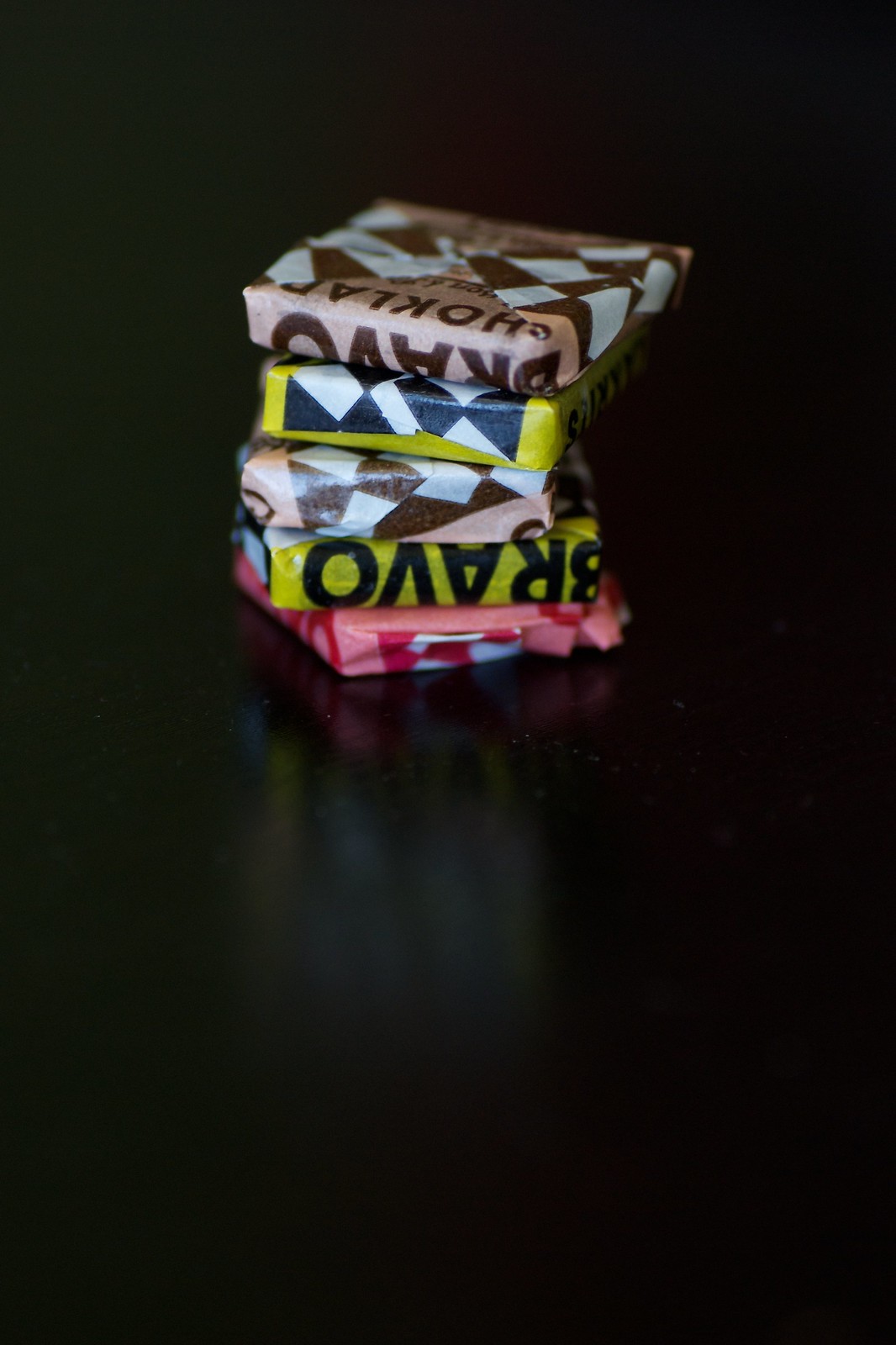The image displays a stack of five packages, possibly bars of chocolate, each wrapped in colorful paper set against a smooth, reflective black surface. The arrangement is almost centered, suggesting an indoor setting, perhaps a kitchen. The packages have various designs involving checkerboard patterns and multiple colors like black, white, brown, tan, yellow, pink, and red. The top package features a checkerboard pattern in brown and white with partial text, "Bravo" and "H-O-K-L-A." Below it, the next package is yellow with a black and white checkerboard design. The following packages include a dark brown one with a similar checkerboard pattern and another yellow one also labeled "Bravo." The bottommost package shows some red and pink. The precise reflective quality of the surface beneath emphasizes the vibrant colors and patterns of the wrappers.